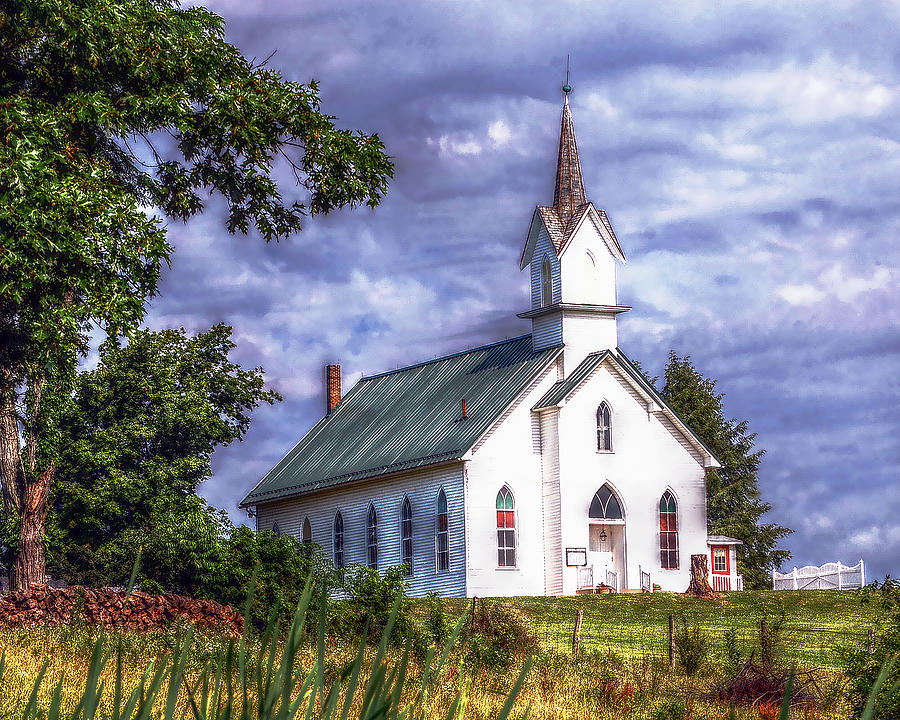This landscape-oriented image appears to be a stylized or semi-illustrated photograph of a white church situated in a rural area. The church features a steeply slanted green roof, which appears somewhat grayish-blue in certain light, and a tall steeple topped with a small blue ball. A brick chimney protrudes from the back of the building. The entrance of the church, located on the right side, includes a pointed arched door, complemented by similar slender arched windows that surround the structure. 

In the scene, the church stands as the solitary building, enveloped by lush greenery. To the right of the church, there is a white picket fence and an additional fence is visible closer to the vantage point of the image. The grassy expanse extends in front of the church, while older, larger trees populate the left side of the scene. Adjacent to the church on the right, a smaller tree can be seen. The sky overhead is cloudy, yet retains a hint of sunlight, casting a natural, serene ambiance.